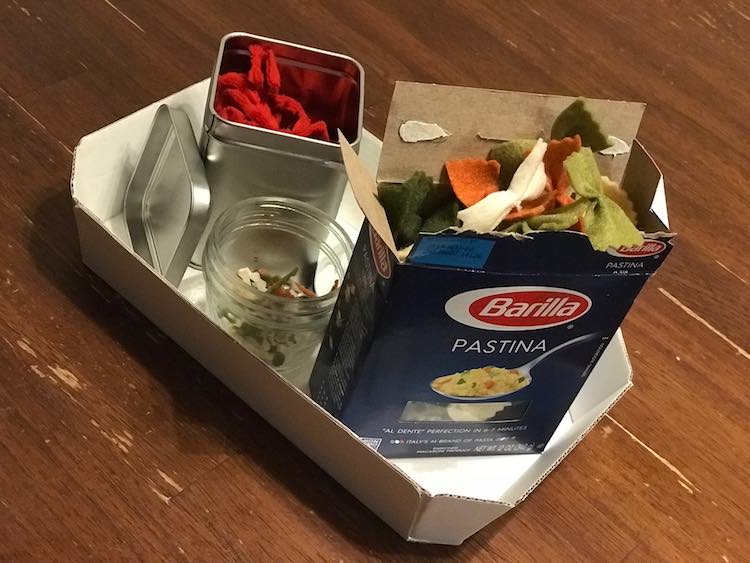The image displays a unique scene with various intriguing objects. Central to the arrangement is a white cardboard box or lid, notably distinguished by its angled corners. Inside this box sits a silver metal tin, possibly containing spices or potpourri. Beside the tin is a small, open jar, approximately pint-sized, which appears to have a screw-on lid mechanism. Its contents are ambiguous, potentially spices or paper.

Adding to the eccentric assortment is a box of Barilla Pastina, conspicuously out of place as it contains what looks like bow-tie pasta. However, upon closer inspection, the bow-ties appear to be intricately crafted from felt, mimicking pasta shapes and colored to resemble spinach, egg, and tomato variants. This felt pasta hints at the likelihood of all the items being pretend food rather than the real thing.

The entire collection is set atop a well-worn wooden table, adding a rustic charm to the overall scene.